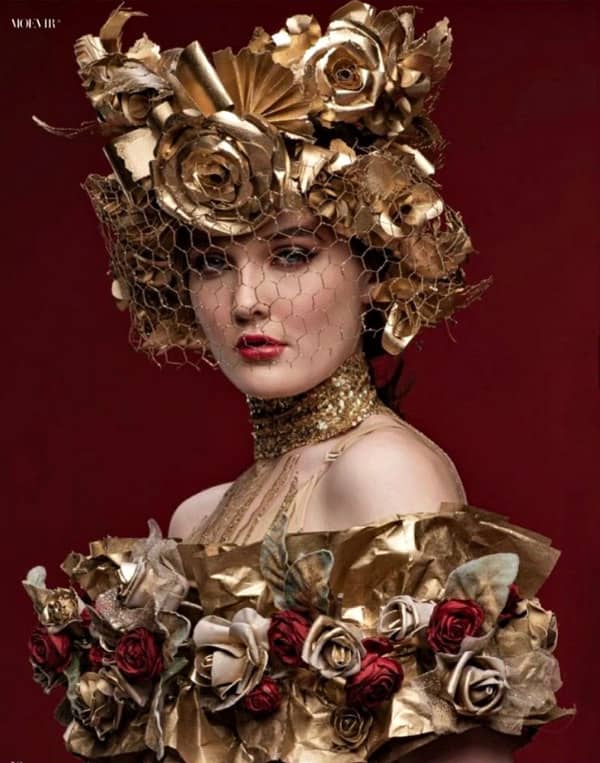The image is a professionally taken photograph of a woman, featuring a detailed and elaborate outfit. She is dressed in a shimmering, metallic gold off-the-shoulder dress adorned with an intricate arrangement of red, white, and gold roses, as well as various folds and frills. The dress, appearing to be made from gold ribbon, has intricate floral patterns, complemented by a series of gold threads extending from her chest area to her gold choker. Her headdress is a strikingly large and elaborate piece, composed of gold roses and abstract shapes, and is veiled with a net featuring hexagonal interlinking patterns that drape down over her face. The woman, who has dark hair and blue eyes, is pictured against a red background with some text visible at the top left. She is viewed from the waist up, and her makeup includes red lipstick, enhancing the elegance of her overall look.